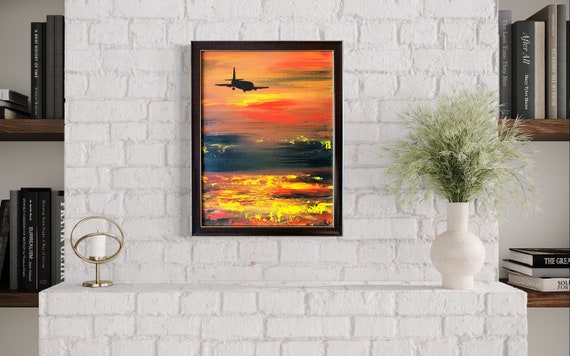This digital photograph, potentially enhanced in Photoshop or professionally edited, captures an elegant brick mantle that has been painted white. Adorning the mantle on the left side is a circular brass game object, adding a touch of vintage charm. On the right side sits a white vase filled with decorative leaves or brush, contrasting gently with the surroundings. The mantle is flanked by two built-in bookshelves on each side, creating a symmetrical and balanced backdrop.

The focal point of the image is a striking, colorful framed painting that occupies a slightly left-of-center position. The painting vividly depicts an ocean scene with the dramatic silhouette of a helicopter set against a fiery orange and yellow sky, encased in a sleek black frame. The photograph is expertly lit, highlighting the details and textures, ensuring a professional and polished presentation.